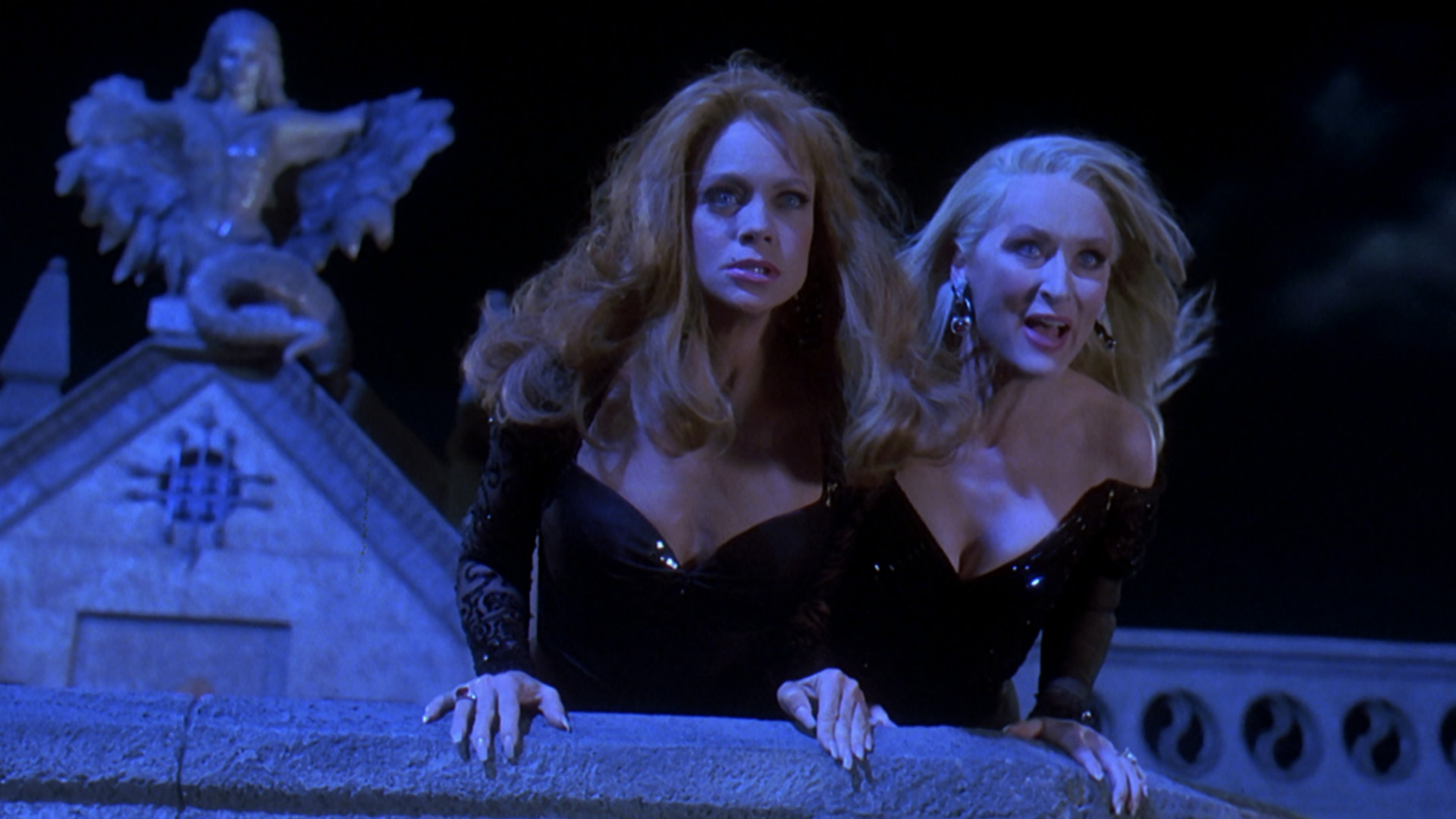In this screenshot from a movie scene, two women stand closely together on the top of a house, specifically on a widow's or crow's nest balcony made of brick with a small retaining fence. The atmosphere is enveloped in a strong blue light, which adds a dramatic, nighttime effect with a fierce, cloudy sky in the background. Both women are dressed in long-sleeved black dresses, with lace detailing, reminiscent of ballroom gowns. The woman on the left has long red hair flowing past her shoulders and strikingly light blue eyes, while the slightly older woman on the right sports blonde hair, the same light blue eyes, and gold earrings. They both appear agitated, staring intensely over the balustrade. Behind them, near the peak of the roof, stands a statue of an angel. The left side of the frame also reveals another statue on an arched roof, further contributing to the gothic, potentially vampire-themed atmosphere of the scene.